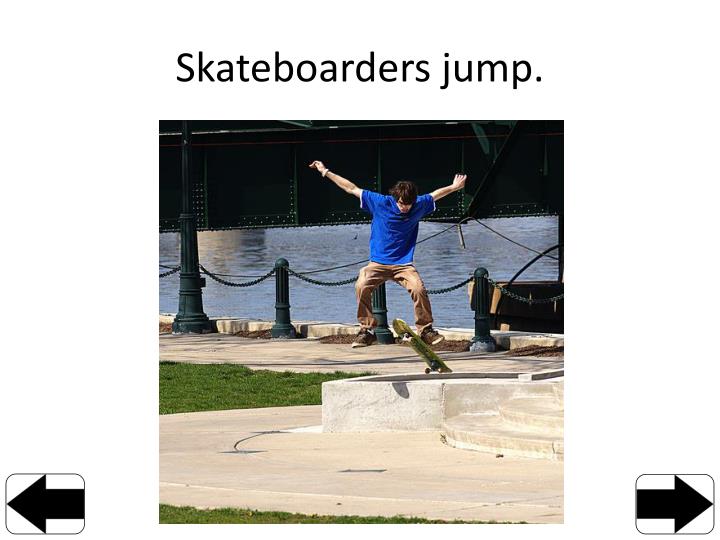The photograph captures a skateboarder mid-air performing a trick known as an ollie over a short concrete wall around 1 to 1.5 feet high. The skateboarder, a light-skinned male with dark hair, is dressed in a blue t-shirt, khaki (or brown) pants, and brown sneakers with white bottoms. His arms are extended out to the sides, and he appears focused, looking down at the skateboard. The skateboard itself is green, with the rear wheels positioned on top of the wall. The surrounding setting includes a concrete plaza with some grass, a sidewalk, and a pier with chains and green-colored posts leading towards a dark body of water in the background, which could be a river. There is a lamppost on the left-hand side of the image. The photograph is featured as part of a slideshow, with black arrows within rounded rectangles on either side, and a title above the image in black text that reads, "Skateboarder's Jump."